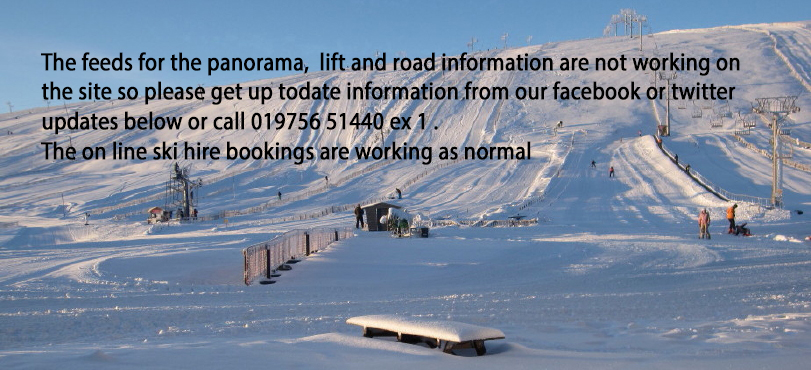The image is a panoramic view of a bustling ski resort area, featuring a large, snowy hill marked by multiple tracked vehicle and ski trails. There are about five distinct lanes, each defined with fences or railings for safety. To the right, a ski lift comprised of wires extending from several Y-shaped metal poles ascends the hill, transporting skiers. The left part of the image showcases a small shack with a man standing next to it, and nearby, a bench rests against the snowy backdrop. Scattered groups of people can be seen skiing down the hill and gathering at the bottom of the slope. The image is bathed in bright sunshine, with a clear blue sky occupying the upper half, creating a vibrant winter scene. Superimposed in the top left corner of the image are four lines of black text stating: "The feeds for the panorama, lift, and road information are not working on the site, so please get up-to-date information from our Facebook or Twitter updates below, or call 01975 651440, extension 1. The online ski hire bookings are working as normal."